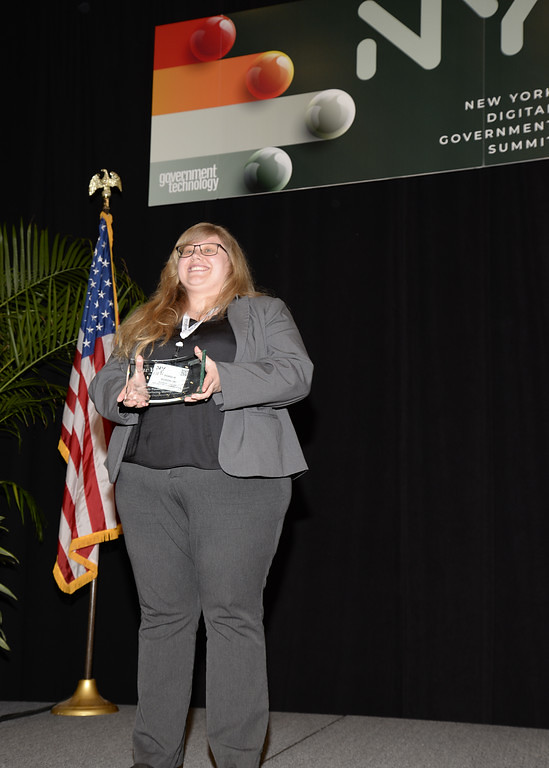The photograph features a woman in her mid to late 20s, standing on a stage and smiling as she holds an award in her hands. She is positioned slightly left of center, wearing a gray suit jacket over a black blouse, paired with gray pants. The woman, who has long reddish-blonde hair and wears black-framed glasses, is facing forward but turned slightly to the left, looking towards another camera outside of the image frame. She appears to be on the heavier side, around 200 pounds. An American flag stands to her left. Above her, a partial banner reads "New York Digital Government Summit" with "Government Technology" visible in the lower left corner, indicating the event at which she is likely accepting the award.